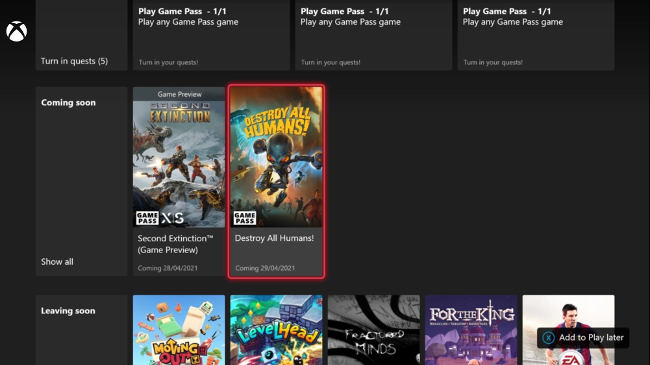This cropped screenshot showcases the Xbox home screen, dominated by a black background. In the top left corner, the iconic white Xbox logo is displayed. Four truncated boxes appear at the top, suggesting the screen has been scrolled down slightly. The first visible box at the bottom contains the text "Turn in quests" accompanied by the number '(5)'. To its right, an advertisement urging users to "Play Game Pass" is prominently positioned. Following this, three additional boxes also encourage engaging with "Play Game Pass," labeled identically as "Play Game Pass 1 of 1."

At the bottom left corner of the screen, the grey text "Turn in your quests" is displayed. Centrally located, the second row begins with a box labeled "Coming Soon" at the top left, with a "Show All" prompt at the bottom. This row features two game thumbnails: "Second Extinction" and "Destroy All Humans," each marked with the Game Pass logo in the bottom left. Notably, "Destroy All Humans" is highlighted with a red box, indicating it is currently selected. The screenshot was captured with the intent to showcase the game "Destroy All Humans" to someone.